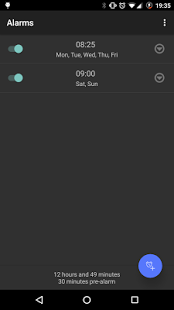The image depicts a blurry cell phone screen with black background and white text. The screen shows alarm settings, indicating that it is 19:35. The status bar at the top displays cell signal bars, a Wi-Fi indicator, and the alarm icon on the left.

Under the "Alarms" header on the top left, two alarms are set. The first alarm is set for 08:25 on weekdays (Monday, Tuesday, Wednesday, Thursday, Friday), and the second alarm is set for 09:00 on weekends (Saturday and Sunday). Both alarms are activated, indicated by turquoise toggles.

Below the alarms, the text reads "12 hours and 49 minutes," signifying the time remaining until the next alarm, and "30 minutes pre-alarm," which likely indicates a pre-alarm setting. 

In the bottom right corner, there is a blue circle with plus and alarm icons, suggesting an option to add a new alarm. The navigation bar at the bottom includes three white icons outlined against a black background: a back arrow, a circle, and a square.

To the right of each alarm, a down-pointing caret in a circle allows for further options or collapse. The image itself is quite blurry with poor resolution, making the text and icons readable but not clear.